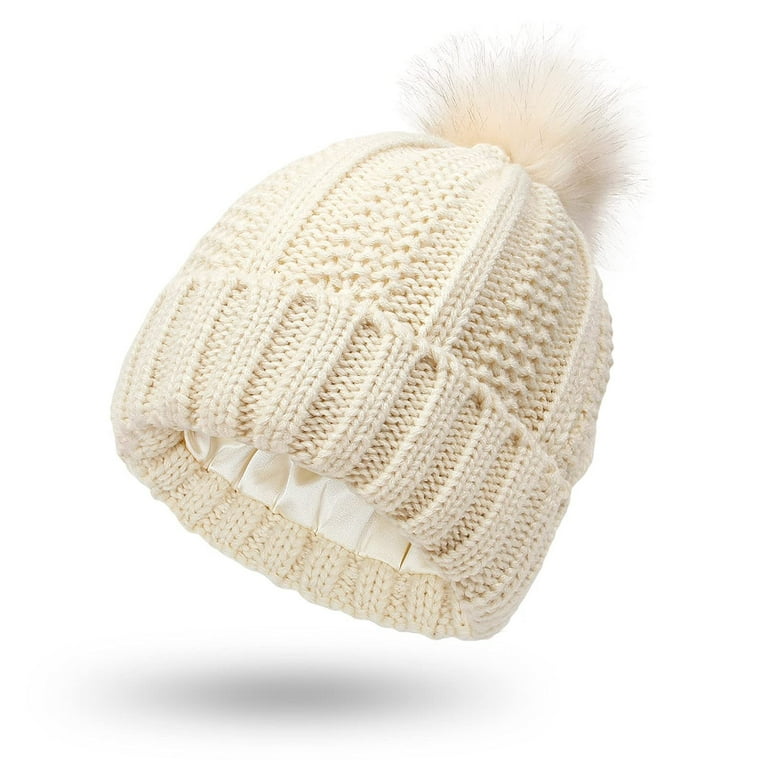This close-up image showcases a beautifully crafted winter beanie hat, prominently centered against a plain white background that highlights its details. The hat, appearing to float and casting a slight shadow beneath, is made from intricately knitted yarn in soft cream and off-white tones. The pattern features vertical lines running from the top to the bottom, culminating in a large, fluffy pom-pom made of fur situated at the top end. The hat's opening, tilted slightly to the left, reveals an interior that is lined with a soft, silky, white material, resembling velvet, which enhances its warmth and comfort. The meticulous knitting includes a few inches of a different design at the base, adding to its handmade charm and overall intricate appearance.